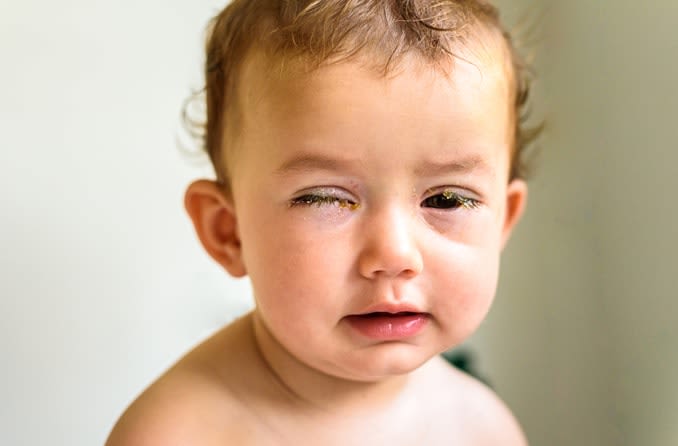The image is an up-close, colored photograph of a young child, likely between 1 and 18 months old. The baby has light skin, dark brown hair with slight waves, and dark eyebrows. His left eye is completely closed and has noticeable gunk on the eyelid and eyelashes, potentially indicating an infection. The right eye is partially open, but also has some gunk on the eyelashes. The baby appears uncomfortable, with a mouth slightly turned downward and slightly open. He does not have a shirt on, and the photo only shows up to just past his neck, capturing the upper torso and head prominently. The background is grayish and somewhat blurred, bringing the focus entirely on the baby. The photograph has an eerie quality, as some elements, particularly around the eyes, seem pixelated or underdeveloped, suggesting the possibility of it being an AI-generated image. The overall expression of the baby is not one of happiness, adding to the unsettling feel of the photograph.